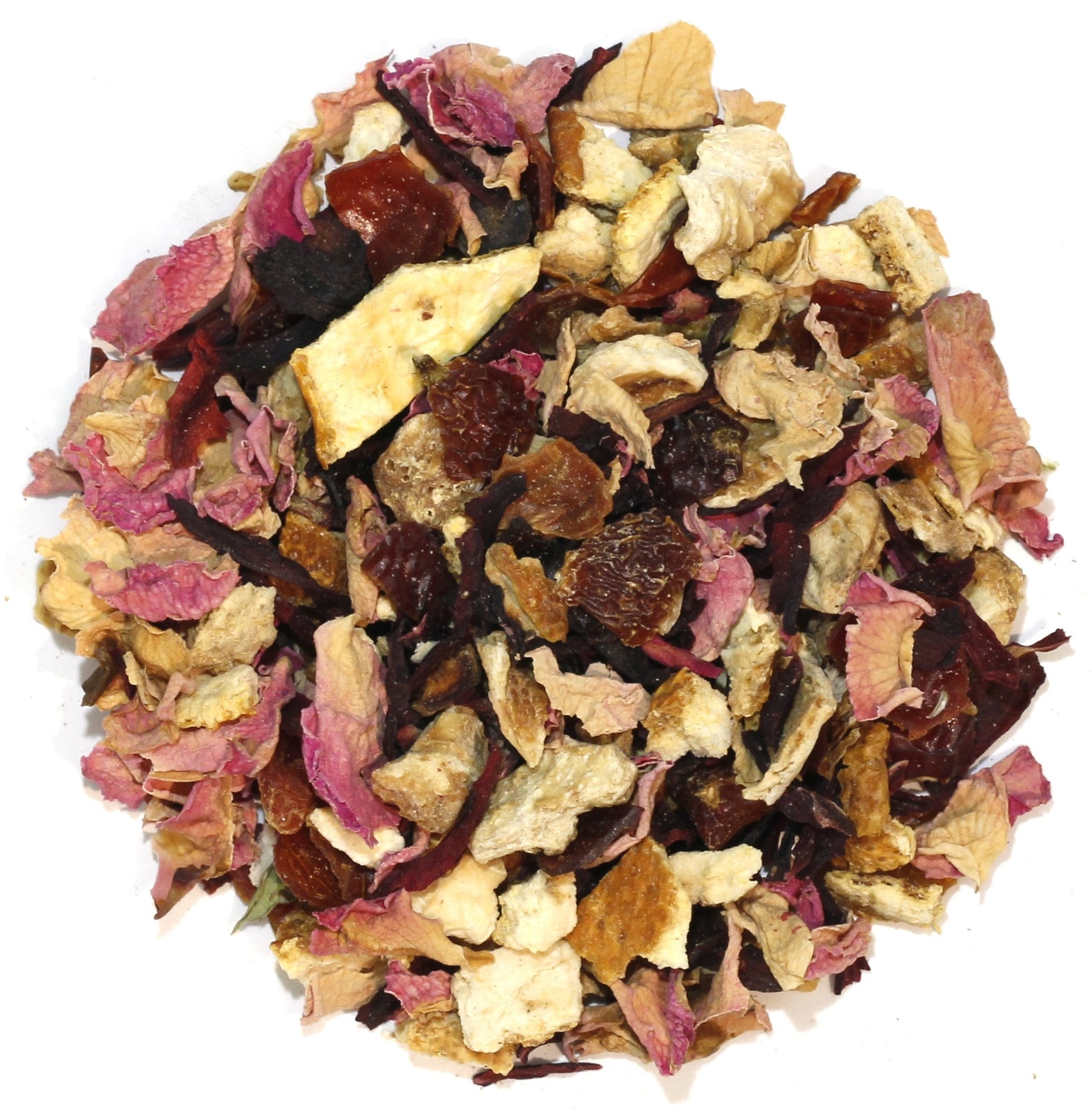This detailed photograph captures an overhead view of a mixed assortment of dried food items arranged in a circular formation against a white background. The various components of the mixture include small, cut pieces of different shapes and colors. Predominantly, there are dry fruits in shades of brown, like dates or raisins, recognized by their wrinkly texture. Among the mix, there are also pieces of light brown or cream-colored items that resemble dried apple sections. Pink and lavender-colored dried flowers add a touch of vibrancy to the array. The overall impression suggests a potpourri-like collection of dried leaves, fruits, and possibly nuts, intricately assembled to form a cohesive, visually appealing cluster.